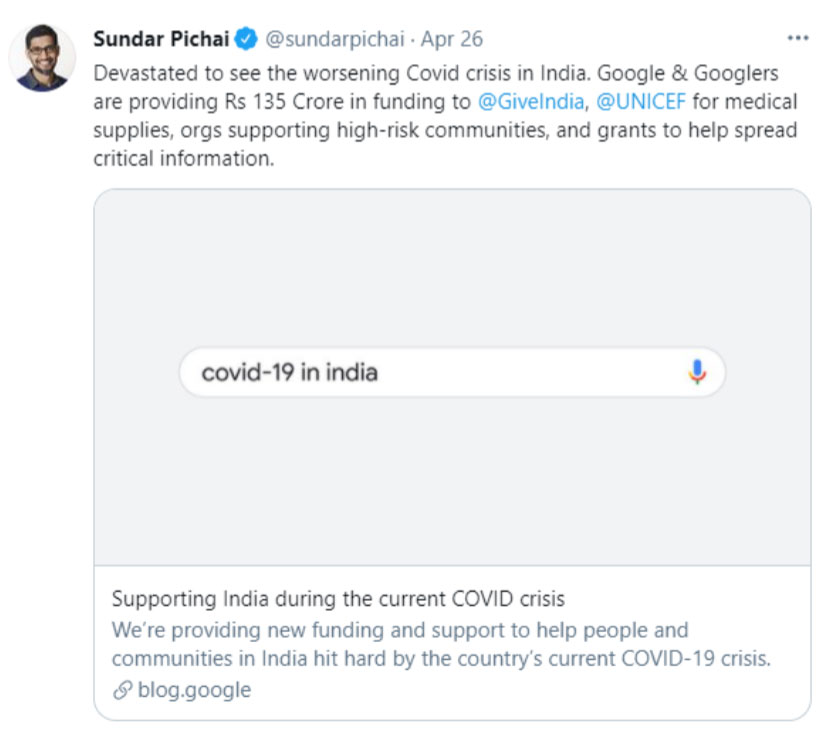The image is slightly taller than it is wide, with a dimension ratio approximately 10-20% taller. In the upper left corner, there is a profile picture of a young man, likely Indian, who has short hair and is wearing glasses and a dark blue collared shirt. This individual is identified as Sundar Pichai, as indicated by the text to the right of the image. Next to his name, there is a blue check mark verifying his identity along with the handle "@sundarpichai" and the date "April 26."

Below his name, there is a tweet which reads: "Devastated to see the worsening COVID crisis in India, Google and Googlers are providing Rs 135 crore in funding to @GiveIndia, @UNICEF for medical supplies, supporting high-risk communities, and grants to help spread critical information."

Below the tweet, there is a search bar displaying the query "COVID-19 in India." Underneath the search bar, there is a paragraph titled "Supporting India During Current COVID Crisis," elaborating on Google's efforts to provide aid and assistance during the pandemic in India.